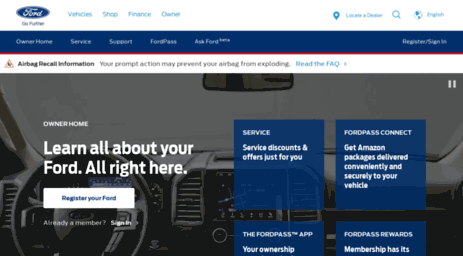The image depicts the homepage of the Ford website, showcasing a detailed and user-friendly interface. In the top left corner, the classic Ford logo is prominently displayed. Adjacent to the logo, several main menu options are visible, including "Vehicles," "Shop," and "Finance," among others. To the top right, a search icon and a dealer locator button are present, facilitating quick navigation.

Beneath the main menu, a conspicuous blue banner with small but legible text features additional headings: "Owner," "Home," "Service," "Support," "FordPass," and "Ask Ford." This banner also includes options for users to register or sign in to their accounts.

Below the blue banner, a white panel provides important information regarding an airbag recall, advising users of a safety recall event affecting specific Ford models.

Dominating the lower portion of the page is a large, immersive image that gives the viewer the sensation of sitting inside a Ford vehicle. The grayscale interior shot highlights the steering wheel and dashboard. To the left of this image, white text reads, "Learn All About Your Ford All Right Here," inviting users to register their Ford vehicles through a button placed underneath this message.

On the right side of the large image, a vertical column of blue panels offers quick access to various services. These include sections for "Servicing," "FordPass Connect," "FordPass App," and "FordPass Rewards," catering to the diverse needs of Ford owners and enthusiasts.